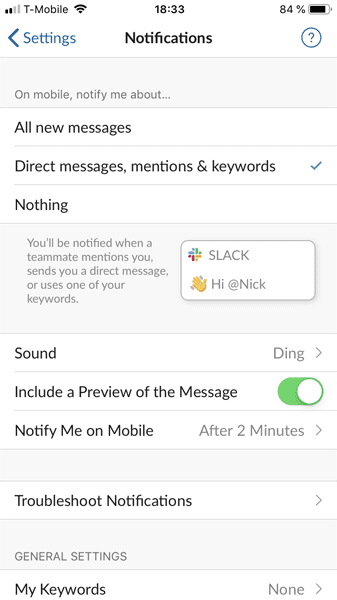This is a detailed screenshot of a smartphone displaying its notifications screen. The background is white, and at the top of the screen, the service carrier "T-Mobile" is visible. The time is shown in military format (24-hour), centered at the top. To the right, the battery percentage is displayed, followed by a battery icon. The title "Notifications" is prominently centered and bold in black at the top of the screen. To its left is a blue "V" shape pointing left, leading to the settings option, and to its right is a blue circle with a question mark inside, indicating help information is available.

Below this header, several notification options are listed. The selected option displays "Direct Messages, Mentions, and Keywords." Just beneath this, a small box with the Slack logo and a waving hand emoji greets the user with the message "Hi @Nick." The sound notification is set to "Ding," and another blue "V" shape pointing right suggests there are additional settings to configure.

Further down, a green notification bubble appears on the left, with a white circle on the right, stating "Notify me after two minutes on mobile." A dropdown menu provides an option to troubleshoot notifications and manage personal keywords, though no keywords are currently set. Options for further customization are available under another dropdown menu.